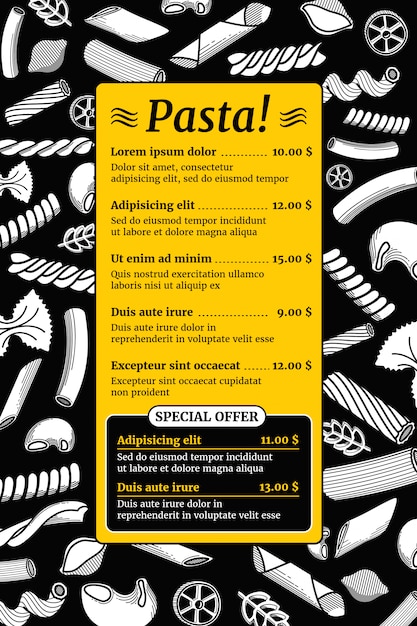This image depicts a stylized restaurant menu in portrait orientation. The background is predominantly black, intricately decorated with graphical representations of various white pasta shapes such as penne, fusilli, wheel-shaped, spiral-shaped, rigatoni, farfalle, and shell pasta, spaced haphazardly around the border. Centrally positioned is a smaller, vertically oriented yellow rectangle which contains the menu text. At the top of this yellow section, "PASTA!" is prominently displayed in black with wavy lines on either side. Below the title, placeholder text including "Lorem Ipsum Dola" represents menu items, followed by a dotted line leading to prices indicated with dollar signs. Each menu item is uniformly spaced and accompanied by two lines of description in non-bold text. The footer of the menu features a black box with a white oval at the top, boldly labeled "SPECIAL OFFER." This section includes placeholders for two special offer items, identified with yellow text and accompanied by descriptions in white text on a black background. Prices for these offerings are also in American currency, indicating a $11 and $13 option. Despite using placeholder text, the detailed design suggests a sophisticated, visually appealing menu template.